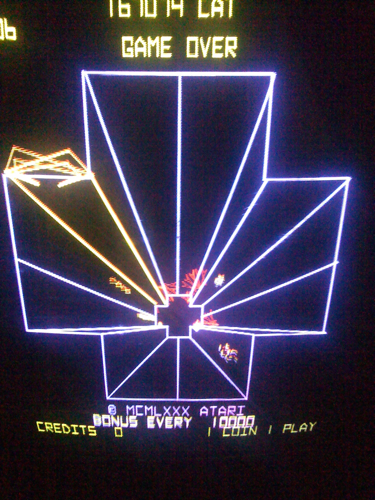The image depicts a still from an older arcade video game screen, characterized by bright, glowing graphics against a dark purplish-black background. At the top of the screen, neon letters display "161079LAT," and just below it, prominently lit in yellow, is the message "Game Over." An intricate three-dimensional design dominates the lower portion of the screen, resembling a cross that is wider at the top and tapers down towards the center. This cross-like structure is outlined in blue and white, with additional illuminating triangular shapes on either side, creating an abstract geometric pattern. Red and yellow lights accent certain parts of the design, adding to its vivid appearance. The bottom of the screen features the text "MCMLXXX Atari" along with "bonus every 10,000 credits," "credit zero," and "one coin play," clearly indicating that it's an end-of-game message from an Atari arcade game, highlighting the era with the MCMLXXX (1980) Roman numerals.